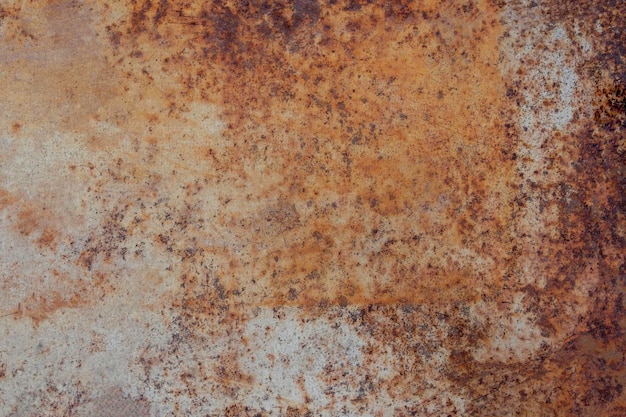This image captures a richly textured, aged piece of metal that has undergone significant weathering. The surface is patinaed with rust, presenting a mesmerizing array of colors and textures. The dominant hues range from a dark brown and black, indicating deep pitting and possibly early stages of corrosion, to gray and silver patches where rust has eaten through, giving the metal a worn, almost decayed appearance. Toward the top and right side, the rust takes on a darker brown shade that gradually fades into an orangish-red center, creating a gradient effect that highlights the metal's aging process. The piece has numerous dark splotches and spots, adding an intricate pattern that resembles an abstract painting. The entire composition evokes imagery of neglected industrial materials, such as an old ship’s hull or a discarded sheet of tin, bringing forth an evocative sense of history and decay.